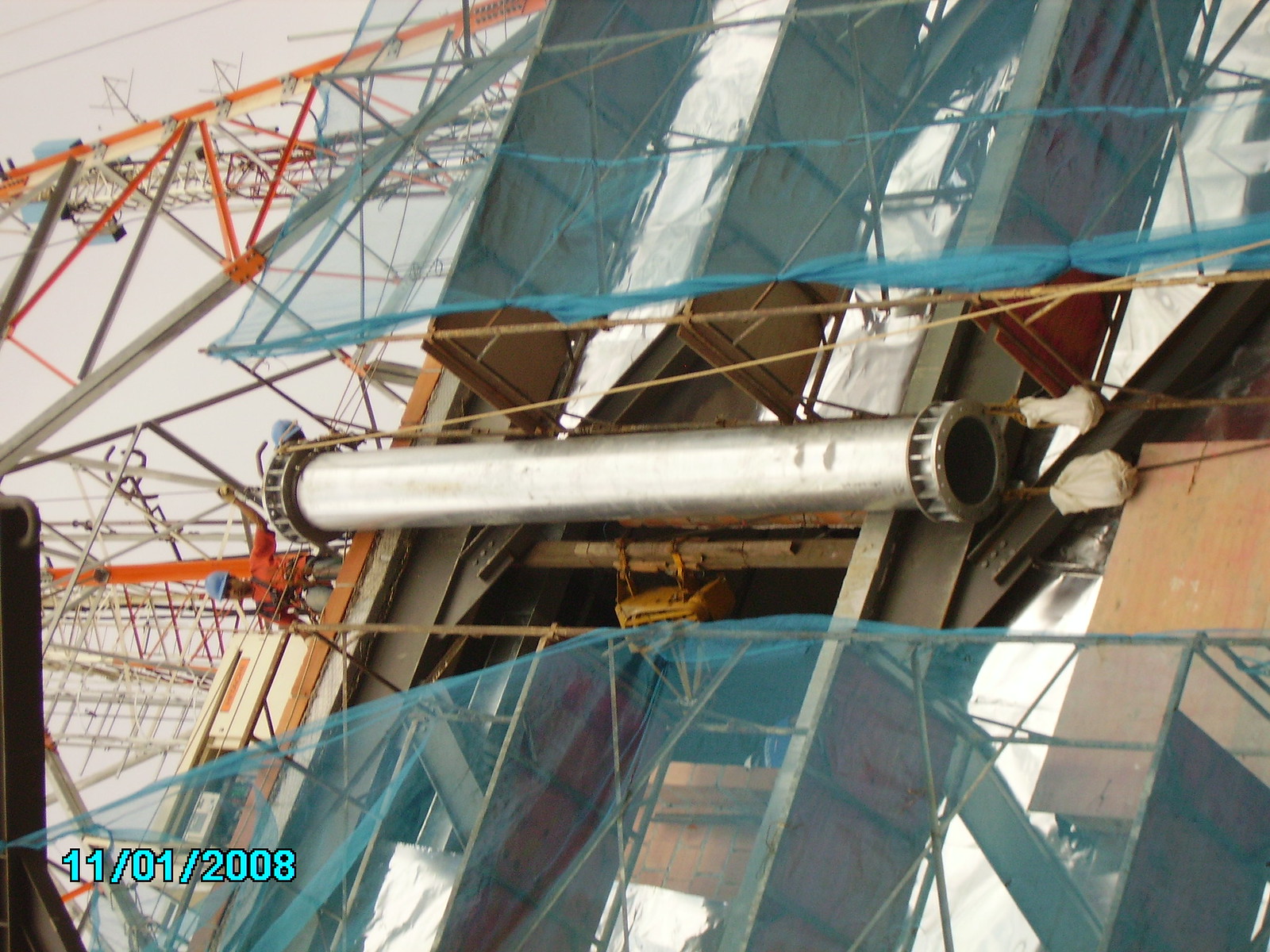The image appears to be a screenshot from security footage taken on November 1, 2008, as indicated by a neon blue date watermark in the lower left-hand corner. The scene depicts a chaotic construction site, potentially a bridge or a building mid-construction, featuring various elements such as a prominent crane and a large pipe likely intended for pouring cement. Blue mesh netting is visible, presumably installed to prevent objects from falling onto pedestrians below. Additionally, some areas are covered with plastic sheets, possibly to protect construction materials from the weather. Two workers can be seen standing atop a steel structure amidst the metal frameworks and wiring, encapsulating the industrious yet disordered nature of the site.